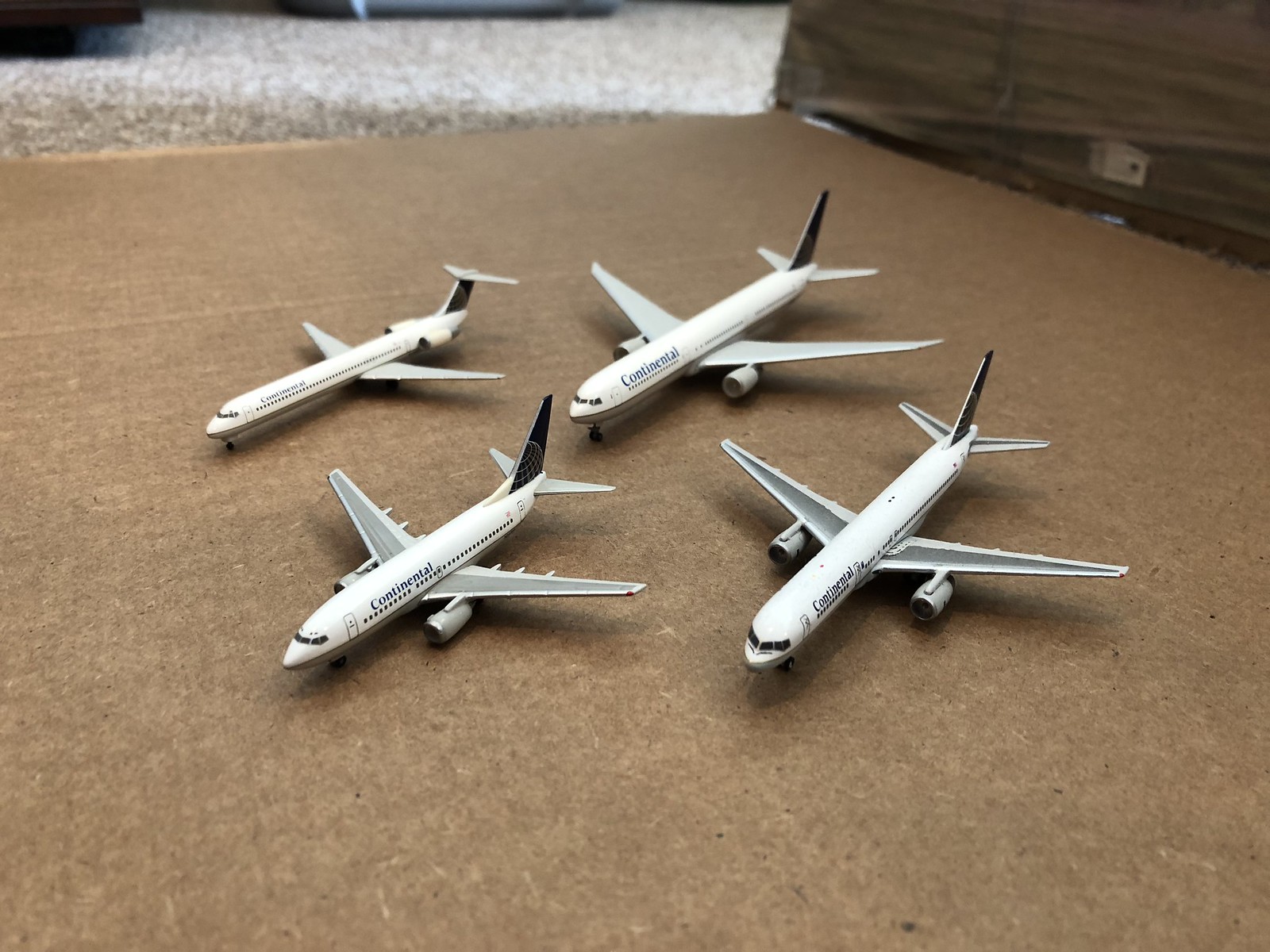This photo shows four small toy planes arranged on a flat surface, most likely a compressed cardboard or paperboard, which is a dark brown color. The planes are aligned towards the bottom left of the image. Each plane features the familiar Continental Airlines livery, characterized by white bodies, dark gray wing tops, and black tails adorned with a white globe design. The planes appear to be models of different aircraft, each with slightly varied wing shapes. Surrounding the planes, the background includes a speckled gray, black, and white surface, possibly carpeting or a counter, and a brown wall panel with some cords visible in the right corner. The combination of these distinct elements suggests a nostalgic setup, possibly implying that the photo predates Continental Airlines' merger with United Airlines.